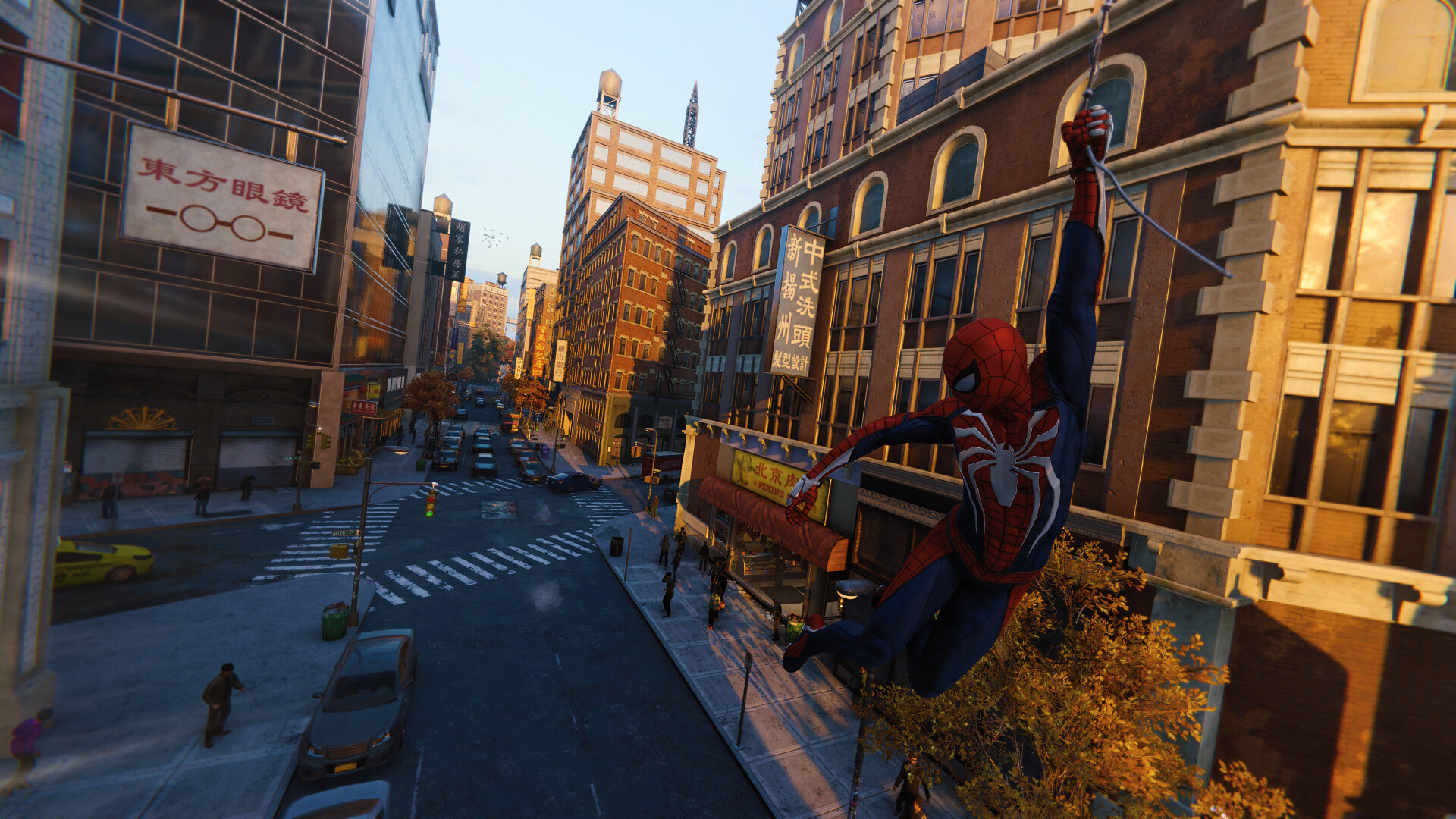In this highly detailed and lifelike screenshot from a Spider-Man video game, the scene captures the vibrant essence of a bustling downtown metropolis. Central to the image is Spider-Man, clad in his iconic red and blue suit adorned with a prominent white spider emblem on his chest. He is positioned on the right third of the image, gripping one of his webs in his left hand as he swings through the city, turning his head to look over his right shoulder. His dynamic pose shows his legs trailing behind him, and we catch a glimpse of only his left eye through the mask.

The urban landscape around him features tall commercial buildings and office blocks on both sides, creating a canyon of architecture through which Spider-Man navigates. On the left side, a glass and steel building contrasts with the brown buildings with numerous windows on the right. Further down this right side, another brown building is visible, indicating the density of the area. A pair of eyeglasses is depicted on a sign attached to one of these buildings, hinting at a retail or optician’s store below.

Traffic is part of the tableau, with a yellow cab emerging from a street on the left and more vehicles lined up at intersections and parked along the sides. The dark gray road features white crosswalk lines, adding to the meticulous urban detail. Despite the numerous elements, the clear blue sky above suggests a bright day in this animated cityscape. The scene depicts the essence of an 'urban jungle,' emphasizing the concrete nature of the environment with just a single tree visible amidst the sidewalks and dense infrastructure. This composite image brilliantly captures the thrilling and intricate world of Spider-Man swinging through a vibrant, digitally-rendered city.